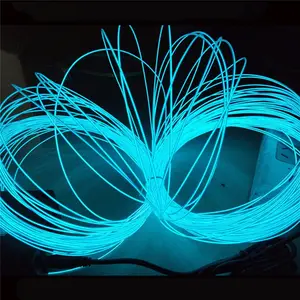The image is a perfectly square photograph set against a pitch-black background, featuring a central object that resembles a vibrant, neon blue slinky. This slinky-like structure is composed of extremely thin, glowing lines that form a semi-circle extending from the left to the right. Due to its high luminosity, the lines appear more condensed and thicker where they overlap on the left and right edges, while they are thinner and more distinguishable towards the center arc. The neon fluorescence of the blue lines resembles the effect seen under a black light, creating a visually striking contrast against the dark backdrop. There are no other elements, text, or colors in the image, ensuring the focus remains solely on the glowing semi-circular formation. The image is crisp, possibly implying it is digitally rendered or a high-quality photograph, devoid of any additional objects or distractions.